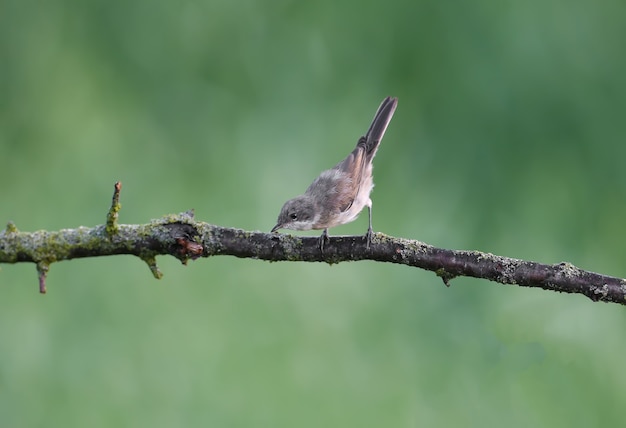The vertical rectangular image captures a serene outdoor scene featuring a small bird perched on a jagged tree branch that extends from left to right across the frame. The background, a blurry blend of various shades of green, suggests a natural environment flushed with trees, brush, and grass. The jagged branch, dark brown to almost black in color, is accented with patches of moss and tiny green twigs. Nestled at the center of the composition, the bird stands diagonally towards the camera but slightly to the left, its dark gray legs and feet gripping the branch. It has a light gray body with a white underside, a darker gray tail, and a small dark gray beak. The beady black eyes are focused downward, giving the impression the bird is either chewing on the branch or inspecting it closely. The close-up framing of the subject against the indistinct green backdrop creates a tranquil and detailed portrayal of nature.